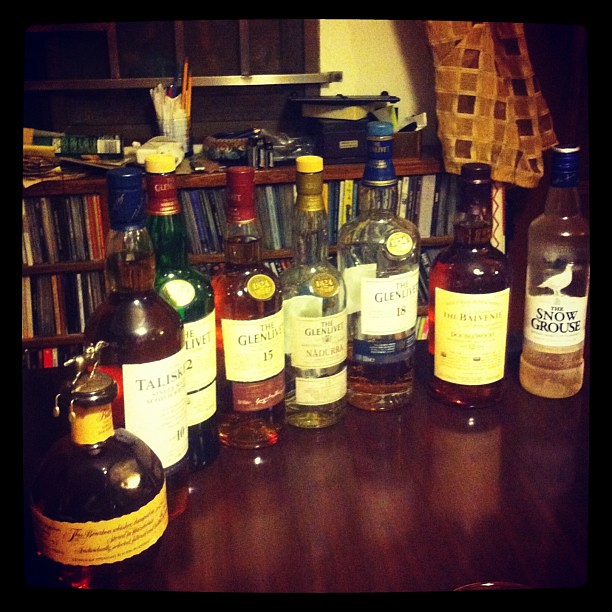The image captures a richly detailed, darkly lit scene of various liquor bottles arranged in a curved row on a shiny, dark wood countertop. The angle is slightly from above, highlighting the assortment of bottles, which include whiskey, vodka, and a significant presence of Glendale scotch in their brown, green, and clear containers. The clear bottles reveal amber liquid inside. Only one label is distinctly visible at the far right, reading "The Snow Grouse," adorned with an image of a bird. The background features an extensive, fully stocked bookcase, adding an intellectual ambiance to the setting. A hint of another piece of furniture is perceptible behind the bookcase, but its details are indeterminate. The overall atmosphere is enhanced by what seems to be a 2013 Instagram filter, adding a nostalgic touch to the scene.